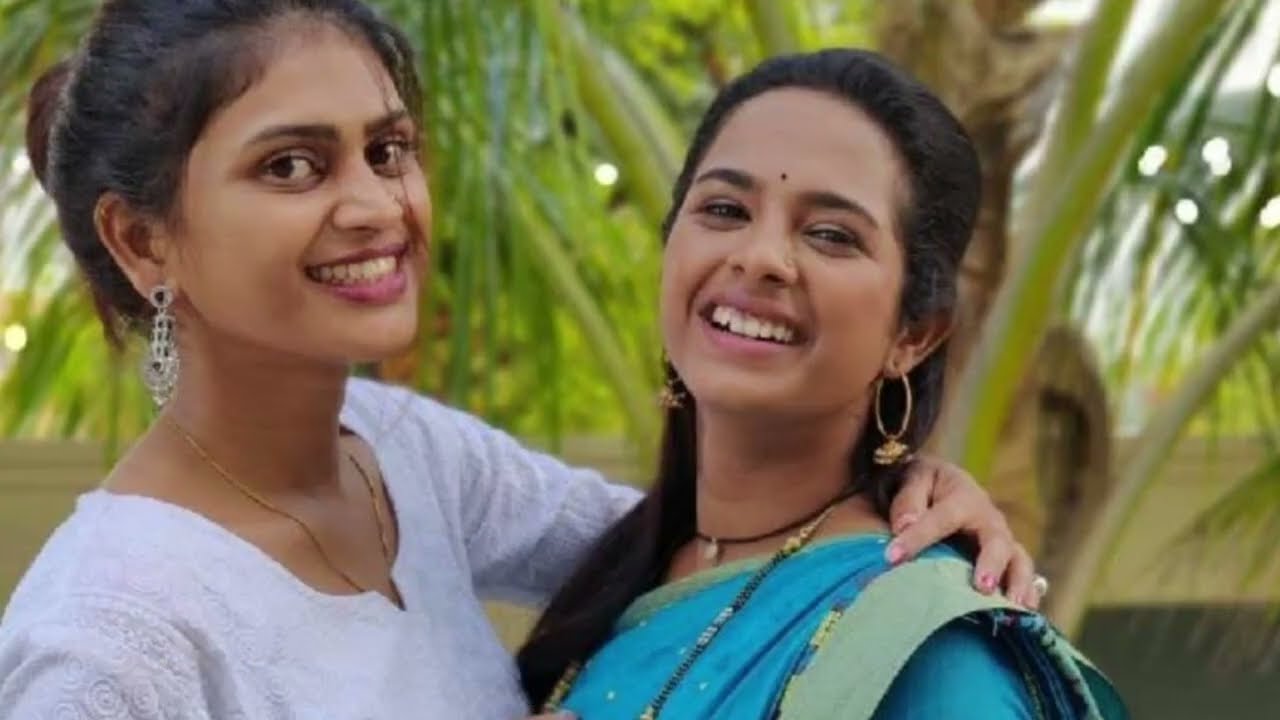This photograph captures two joyful South Asian women, likely Indian, posing outdoors amidst lush tropical foliage. Both women are smiling warmly at the camera, creating a sense of happiness and connection. The woman on the left has her hair pulled back into a bun and is adorned with dangly earrings and a thin gold necklace, wearing an intricately woven white top. She is embracing the woman on the right, who has a bindi on her forehead, gold hoop earrings, and is dressed in a blue and green traditional Indian dress. Her black hair is neatly pulled back. The background features dense, dark leaves, a glimpse of a palm tree trunk, and a brown wall that frames this serene outdoor setting, suggesting a festive or familial gathering in the summertime.